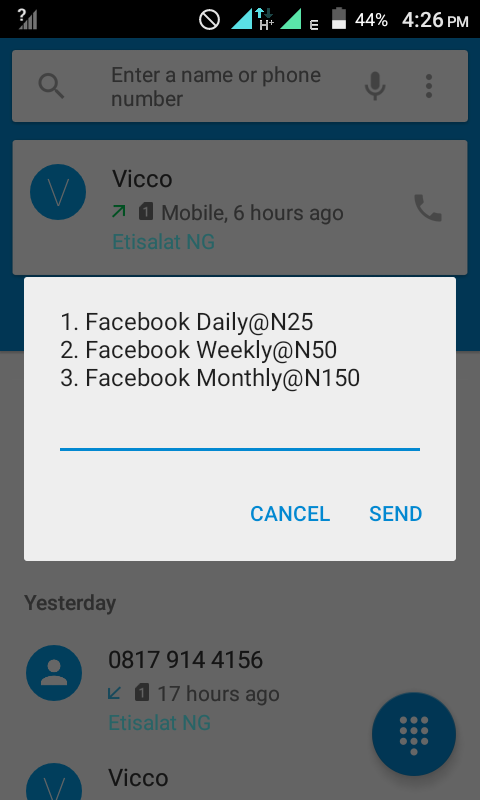A cropped image displays a pop-up message on an older Android phone, suggested by the lower resolution of approximately 720p and the larger black banner at the top. The status bar indicates an EDGE connection—an outdated network type—alongside a full H connection, both symbolized by differently shaded blue icons (one teal, one greenish). The phone shows a 44% battery level with a white icon, and the time as 4:26 PM in white text. A question mark over four bars suggests a non-connected SIM card. 

The background reveals the phone app's recent calls list, grayed out due to the active pop-up. The white-background pop-up is divided by a blue line, separating the "Cancel" and "Send" buttons, also in blue text. The message offers three Facebook data plans: 
1. Facebook Daily at N25.
2. Facebook Weekly at N50.
3. Facebook Monthly at N150.

In the call list behind the pop-up, missed calls are visible: one from a non-US number, and another from a contact labeled "Vico" with a blue "V" icon. To the right, the standard Android number pad icon appears as a blue circle with white buttons.